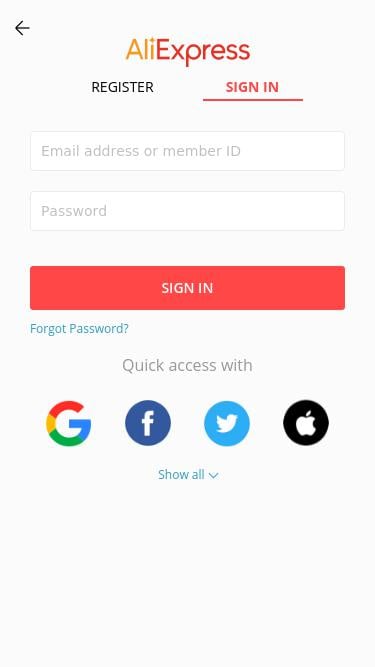A vertical screenshot captured on a narrow cell phone screen displays the login interface for the AliExpress website. At the top of the screenshot, "AliExpress" is prominently featured, with "Ali" in orange font and "Express" in red font, seamlessly attached. Below this header, two options are available: "Register" in black font and "Sign In" in red font. The selected "Sign In" option reveals two text input boxes: one for an email address or member ID and the other for a password. A bright red "Sign In" button, with white font, spans the width of the screen, ready to be tapped. Below this button is the "Forgot Password" link in light blue font. Further down, there are quick access hyperlinks to sign in via Google, Facebook, Twitter, and the Apple Store, with a button to show additional options.